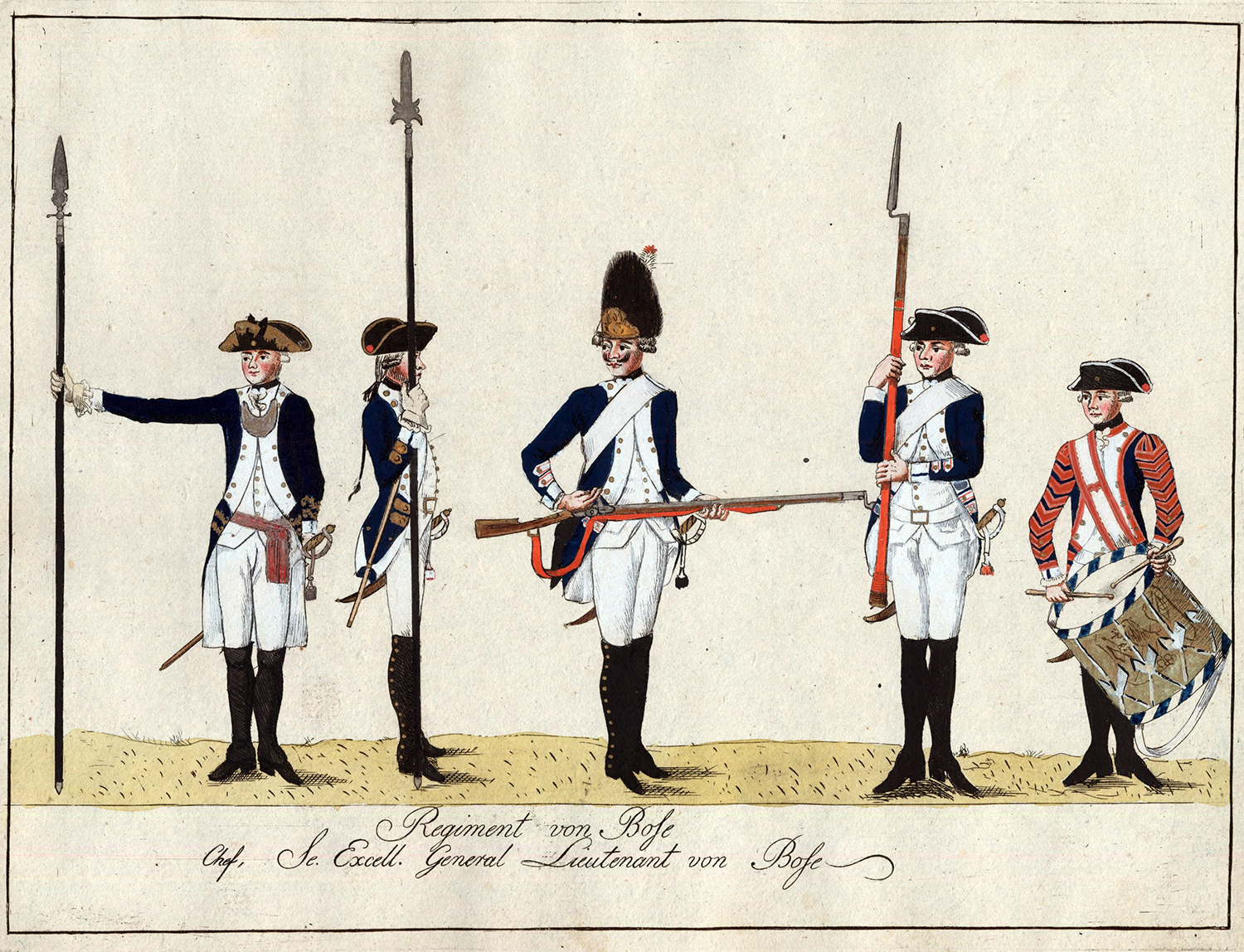The image is a detailed, rectangular drawing depicting five soldiers from an era long past, possibly the Civil War. The background resembles white paper spotted with brown stains, adding a vintage feel. A thin black border lines the edges of the image. Below the soldiers, cursive text reads: "Regiment Von Bull, Chapter E-X-L, General Lieutenant Von Bull."

The soldier on the far right, distinguished by his red jacket and black tricorn hat, holds a drum and drumsticks. Next to him stands a soldier clad in a white uniform with navy blue sleeves, holding a red-colored musket. The remaining soldiers, also dressed in white and navy blue uniforms with long black boots, carry muskets with bayonets. Additionally, the two soldiers on the left hold spears. The central figure, suggested to be General Lieutenant Von Bull, is prominently positioned, commanding attention amidst the troop. Each man wears a distinct black hat, completing their historical military attire.